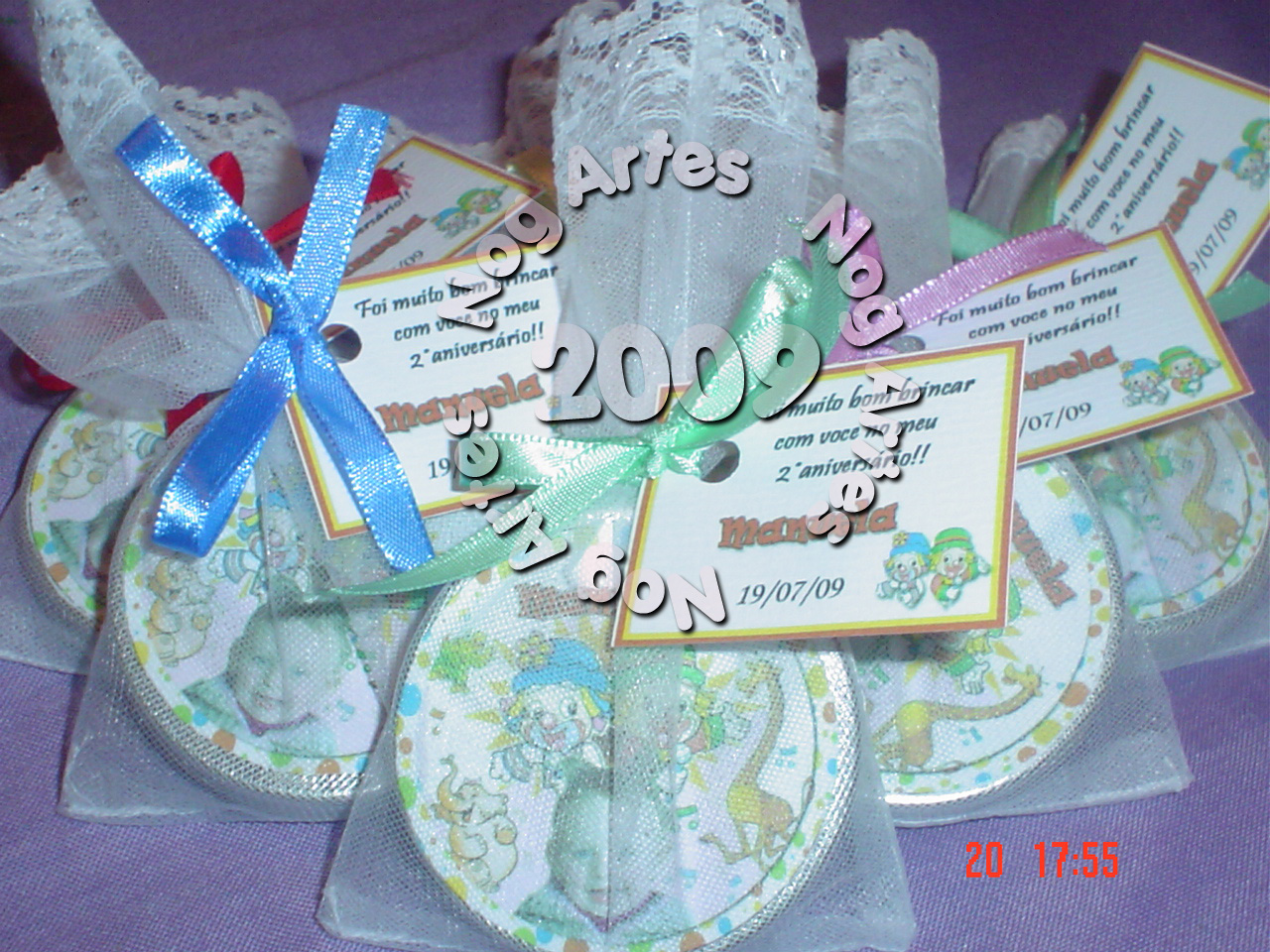This image depicts a collection of party favors designed for a young boy's birthday celebration, possibly his second one. Each favor is enclosed in a see-through mesh bag with lace accents at the top, tied off with colorful ribbons – blue, pink, and green ribbons can be seen. The favors feature an image of a baby boy surrounded by charming cartoon characters such as an elephant, a giraffe, and two clowns, as well as clouds, all set against a white background with multicolored polka dots. Attached to each bag is a paper card, one of which is labeled with the date "19/07/09" and the phrase "2 anniversario," suggesting a special milestone. The favors are branded with "Nog Artists" in a repetitive circular pattern, with "2009" prominently displayed in the center. Additionally, there is a timestamp at the bottom right corner of the photo that reads "20:1755".